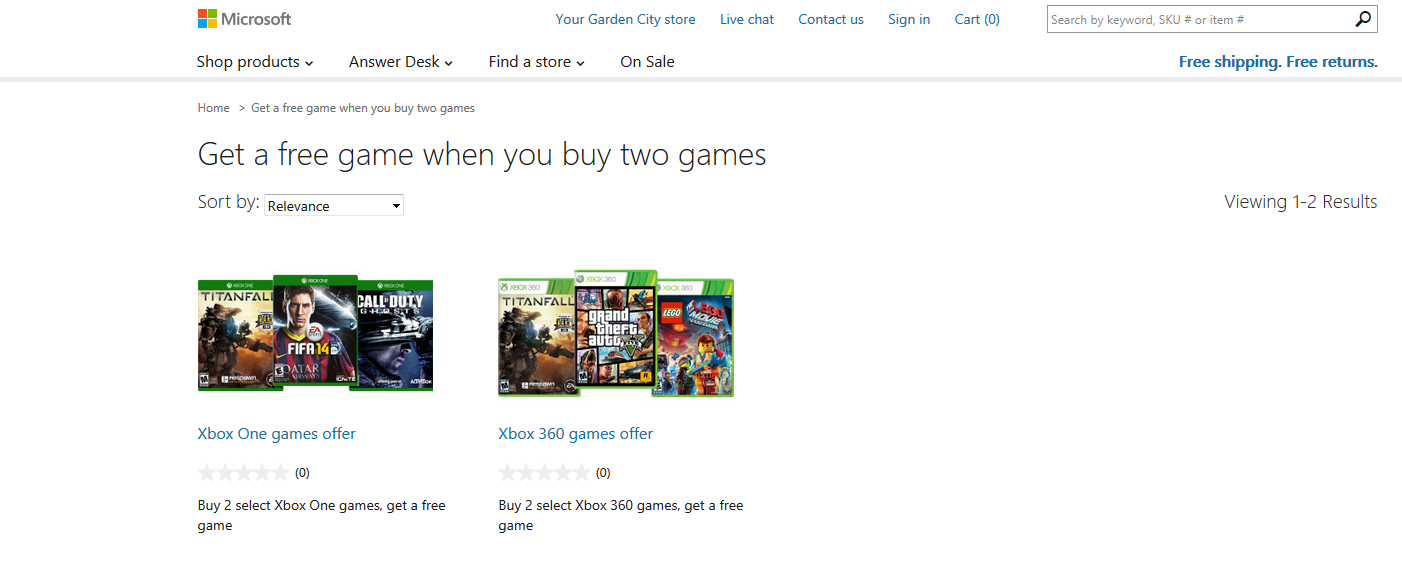Screenshot of the Microsoft Marketplace website with a detailed promotional offer: 

The screenshot features the Microsoft Marketplace website against a pristine white background. At the very top, the header displays various user navigation options including the "Garden City" store location, "Live Chat," "Contact Us," "Sign In," and a cart indicating "(0)" items. To the right of the cart icon is a prominent search bar. Directly beneath the search bar, exclusive customer benefits like "Free Shipping" and "Free Returns" are highlighted.

On the left side of the page under the search bar, a series of navigational tabs—labeled "Shop Products," "Answer Desk," "Find a Store," and "On Sale"—feature drop-down arrows indicating submenus for further options. These are all separated from the main content by a subtle light gray line.

Below this line are breadcrumb links that guide the user’s path; it reads "Home > Get a Free Game When You Buy Two Games." This is followed by a large, bold header stating the same promotional offer: "Get a Free Game When You Buy Two Games."

Directly below the header, a sorting drop-down menu labeled "Sort by" is available, defaulting to "Relevance," and indicates that 1 to 2 results are being viewed. 

The first result listed showcases an offer for Xbox One games with a title "Xbox One Games Offer." This offer currently has no customer reviews—indicated by the lack of highlighted stars—and promotes a deal where customers can buy two select Xbox One games to receive a third game for free.

Next to this, the second result displays an "Xbox 360 Games Offer" with a similar promotion. Though it shows five outlined stars, there are no reviews submitted. This offer also entitles customers to receive a free game when they purchase two selected Xbox 360 games.

This layout is typical of the sales section on the Microsoft Marketplace app or website, designed to showcase current deals on gaming products.